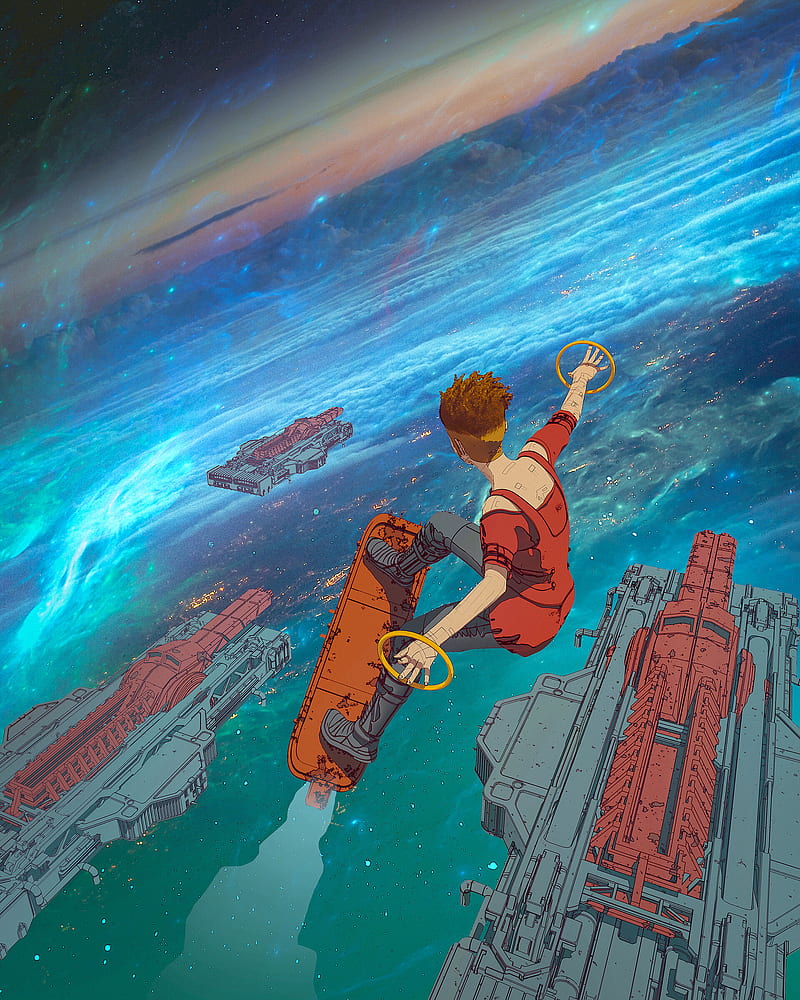The digital artwork depicts a human figure, possibly gender-neutral, with their back turned toward the viewer, air-surfing in what seems to be low orbit or the upper atmosphere of an otherworldly, Earth-like planet. The character is detailed with dark gray pants, gray boots, and a red short-sleeved top. Their hair is tied up in a bandana. They are standing in a semi-squatted stance on a flying skateboard-like device, which even includes a steering wheel. The figure's arms are outstretched, each hand surrounded by two yellow rings, as if guiding their movement through the air. Below them, against a backdrop of turquoise and blue—a palette reminiscent of a planet mixed with aurora borealis-like waves—are multiple large, armored spaceships that bear red and black elements akin to the character's outfit. These military-like vehicles trail beneath the surfer, coasting just above the planet's colorful horizon, adding a definitive futuristic, sci-fi atmosphere to the scene.